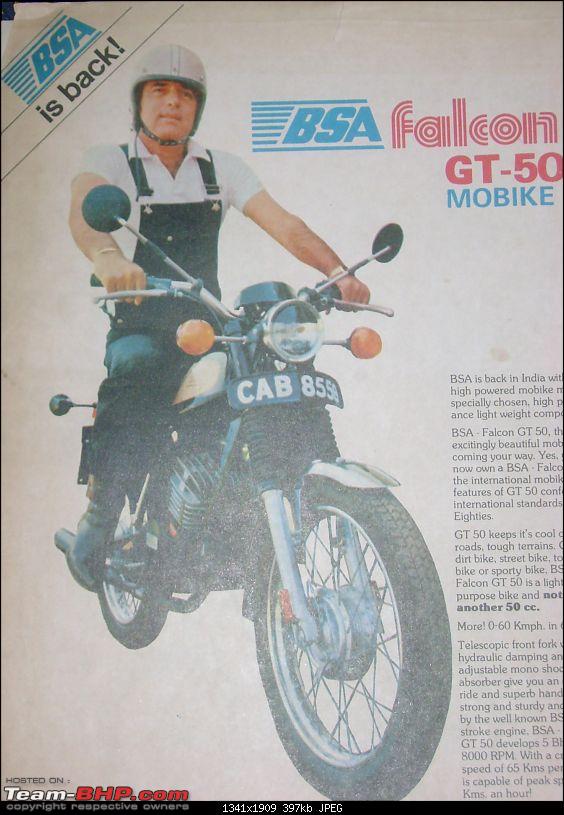The magazine page features prominently a man confidently riding a black moped bike, identified as the BSA Falcon GT50. The rider, wearing a white helmet, a white short-sleeved shirt resembling a polo with a silver apron-like overlay, and black pants, grips the handlebars firmly. The moped's license plate reads CAB 855, with the last digit partly obscured. The upper left corner of the page showcases the bold text "BSA IS BACK," in a diagonal arrangement, emphasizing the resurgence of BSA motorcycles. Below this, the letters "BSA" appear prominently, followed by "ISPAC" in black text. Towards the right edge of the image, another BSA symbol appears, accompanied by the model designation "Falcon GT-50 Moped Bike." The bottom right and center right sections of the page are filled with paragraphs detailing the features and specifications of the motorcycle. In the bottom left corner, there’s a URL: teambhp.com. The overall layout and wording, including the red and blue text, reinforce the advertisement's message about BSA motorcycles' availability and prominence in the market.